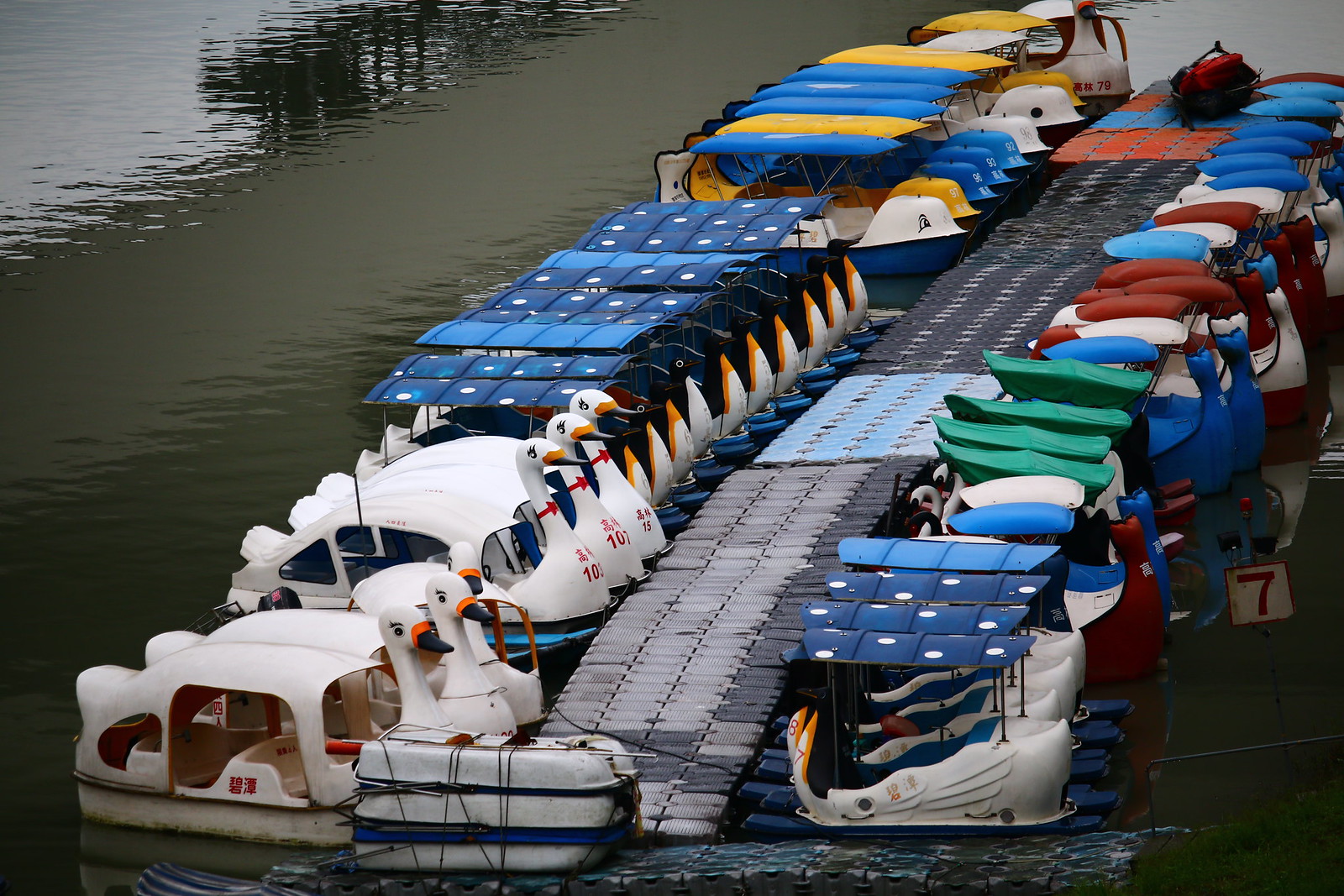The photograph showcases a vivid and playful scene at a floating dock set against a reflective, dark body of water, suggesting a gray, overcast day. The dock itself is a mosaic of interlocking plastic pieces in grays, light blues, reds, and oranges. Lined up meticulously along this floating platform are an array of whimsical paddle boats, each featuring distinct animal themes. To the left of the image, clusters of swan boats with covered seating stand out, their front ends adorned with graceful swan heads. These boats are interspersed with others, like those with penguin motifs, characterized by black, yellow, and white coloring. Beyond these, towards the middle and right areas of the dock, more boats featuring vibrant yellow and blue hues can be observed. There are additional boats with imaginative designs, including ones that resemble whale tails, accompanied by small roofs in shades of blue, red, and white. Altogether, approximately two dozen boats create a colorful spectacle, suggesting an upcoming fun competition or event centered around these charming animal-themed paddle boats.